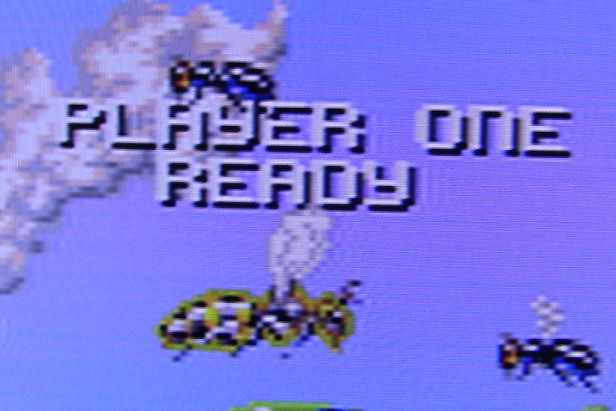The photo in question is a screenshot of an old video game, likely from the early 80s, though it's unclear whether it's an arcade game or a console game. The game's screen displays a blue sky with a couple of white clouds. In the foreground, there are three insects: two are smaller flies, with one positioned at the top and the other at the bottom right of the screen, each having distinct white wings and orangish-red eyes. Dominating the scene is a large bee—possibly a queen bee—noticeable for its yellow and black stripes and white wings, located at the bottom center of the screen. The screen also features text at the top, reading "Player One Ready," indicating the game's preparation for a single player. Additionally, there are hints of green, suggesting plant life, which can be seen at the bottom center and the bottom right corner of the image.